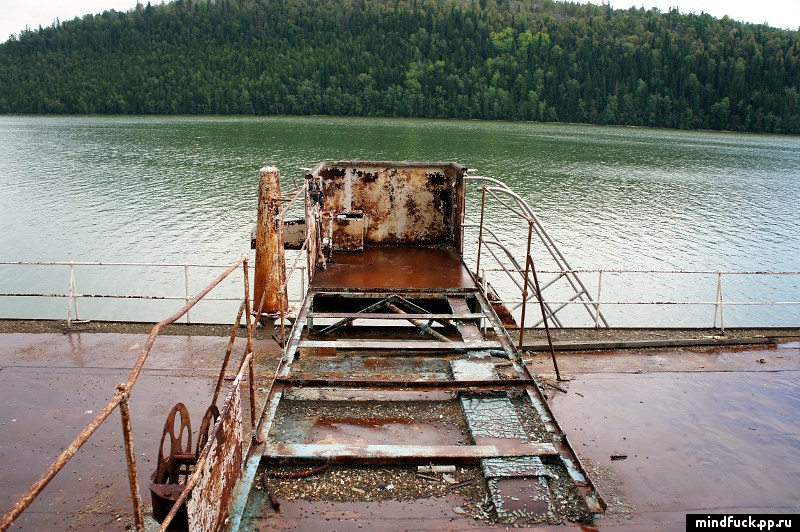The image showcases a large body of water that could either be a lake or a river, stretching out towards a distant, tree-covered hilly region under a glimpse of a white sky during the daytime. The foreground features a vast, rusted, and worn-out metal structure with a brown-colored floor, which likely serves as a viewing platform or the deck of a large, derelict boat. This structure includes a railing on the left and a staircase descending towards the water. The angle of the picture suggests it was taken from this platform. No people are visible in the image. In the bottom right corner, there's a source watermark in a black box with white font that reads "mindfuck.tpr.ru".